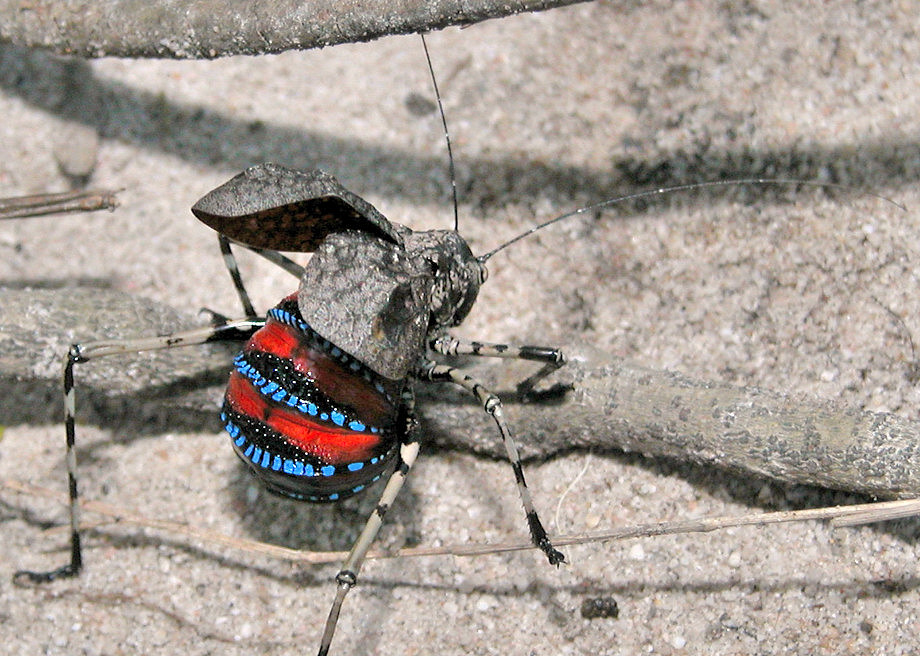This detailed image showcases an intriguing, unidentified insect with a unique blend of characteristics reminiscent of a spider and a cricket. The insect is positioned off-center to the left, crawling on a terrain that appears to be composed of sandy grey and brownish-grey dirt, interspersed with small rock particles and textured sticks. Two prominent sticks run through the scene, casting slight shadows in the daylight.

The insect's body is predominantly black with evenly spaced blue dots and red stripes, providing a vibrant contrast to the muted background. It has a rounded body shape with long, spider-like legs – three on each side – consisting of an off-white color interlaced with black, with the hind legs noticeably longer and angled similarly to those of a cricket. 

The insect's head, which is grey and shiny, resembles that of a grasshopper and gives off a somewhat metallic appearance. It is facing away, obscuring its face, but its two long antennas are prominently displayed. The insect's wings and head, merging into the sandy surroundings, suggest a camouflage adaptation. The focal point remains squarely on this distinctive insect as it navigates across its intricate environment.